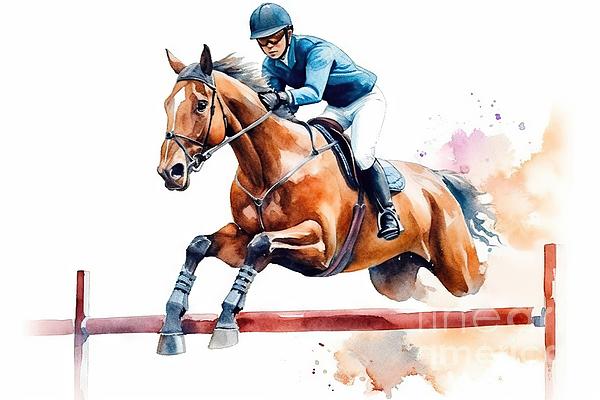The image is a highly detailed watercolor painting of a chestnut-colored horse mid-jump over a red wooden fence on an obstacle course. The horse, showcasing its athletic form, has a distinctive white patch between its eyes, complemented by black ears, a black mane, and a flowing black tail. As it propels forward, you can almost envision its powerful back legs trailing behind. There's a touch of brown watercolor near its hindquarters, suggesting kicked-up mud or dirt from the jump. The rider, standing and leaning forward in a focused pose, is wearing a black helmet with a chin strap and goggles. Their attire includes a blue jacket, white pants, black boots, and gloves, encapsulating typical jockey gear. The background is entirely white, emphasizing the dynamic action and leaving no other contextual elements except the central figures. A partially legible watermark is present on the painting, hinting at an artist's mark.